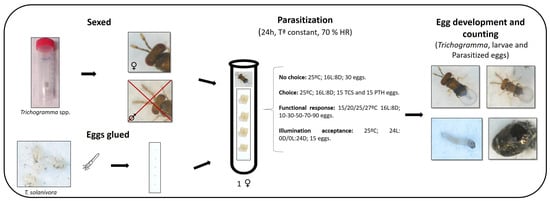This illustration, resembling a page from a biology book, is framed by a horizontal rectangle with a black, thin-lined border and curved corners. On the left, labeled sections "sexed" and "eggs glued" feature images of test tubes and microscopic views of bugs—characterized by dark brown bodies with antennas—along with diagonal red Xs over some insect images. In the center, under the heading "parasitization," there is detailed text mentioning "24 hour T constant" and "70% HR," alongside a vertical bar and images of test tubes containing beige-colored eggs and grayish material. On the right, the section titled "egg development and counting" displays a grid of four stages in the life cycle of trichogramma larvae and parasitized eggs, showing various stages of the larvae and insects in different contexts, including a blue background larvae image and a dark bulb-like object. The diagram, punctuated by black arrows linking the stages, clearly details the developmental process of these parasitic insects.